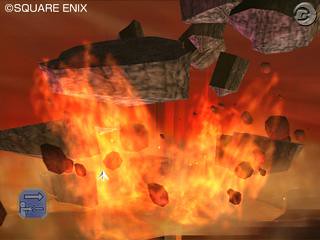A screenshot from a Square Enix video game displays an intense explosion at the center. In the upper left-hand corner, the Square Enix logo appears, preceded by a copyright symbol (©). The lower left-hand portion of the image features a blue square with a right-pointing arrow and an indistinct image, possibly depicting a person.

The explosion in the middle of the frame is vibrant and dynamic, starting with bright yellow hues at the base, which transition into orange and finally darker orange shades as they radiate outward. On the far right, the explosion incorporates red and gray lines, adding to the dramatic effect.

The force of the explosion has shattered a large boulder into several pieces. The largest fragment is seen flying towards the upper left, while other sizable chunks are propelled to the upper right. Smaller debris is scattered throughout the scene, accentuating the chaotic energy of the moment.